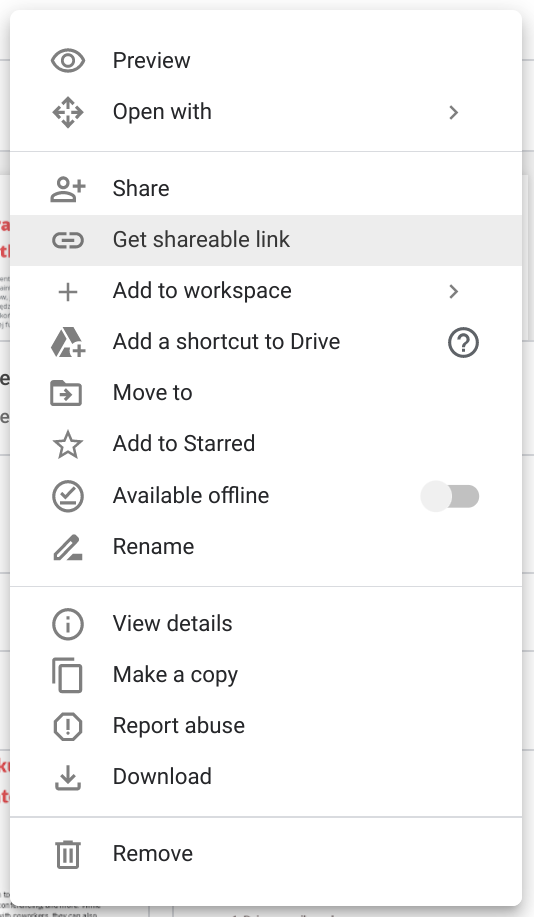**Detailed Description of the Settings Page**

The image depicts a comprehensive settings page on a white background. The settings are organized in a long list as follows:

1. **Preview**: Indicated by an eye icon.
2. **Open with**: This option includes an arrow icon, branching into four separate arrows pointing in different directions.
3. **Share**: Represented by an icon of the top of a person with a plus sign.
4. **Get shareable link**: Denoted by a paperclip icon.
5. **Add to Workspace**: This option has an arrow with a plus sign.
6. **Add to shortcut drive**: Marked by a gray triangle with a plus sign.
7. **Move to**: Displayed with a folder icon and an arrow pointing to the right.
8. **Add to Starred**: Accompanied by a star icon.
9. **Available offline**: This option appears to be turned off and is shown in gray.
10. **Rename**: Represented by a pencil icon.
11. **View details**: Indicated with a circular eye icon.
12. **Make a copy**: Displayed with an icon of a piece of paper.
13. **Report abuse**: Marked by an exclamation mark inside a circle.
14. **Download**: Shown as an underscore with an arrow pointing downward.
15. **Remove**: Represented by a garbage bin icon.